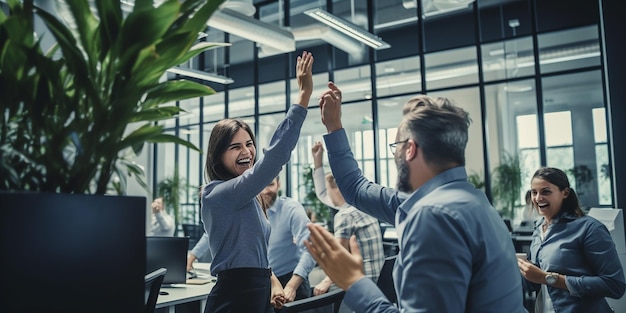In this vibrant office setting, a diverse group of staff members are depicted engaged in a moment of celebration. Dominated by floor-to-ceiling windows that flood the space with natural light, the room features a mix of desks and cubicles, accentuated by light fixtures hanging from the high ceiling and a sprinkling of potted plants that add a touch of greenery to the mostly gray environment. Front and center, a man and a woman, both dressed in light blue collared shirts, are captured mid-high-five, their faces radiating joy and accomplishment. To the right, a woman grins broadly as she observes the high-five, also clad in the similar business attire. Scattered throughout the background, other employees—also in light blue, buttoned-up collared shirts—are engaged in various activities: some are conversing in small groups, others seated at their desks, and a few standing, all contributing to an atmosphere of communal success.